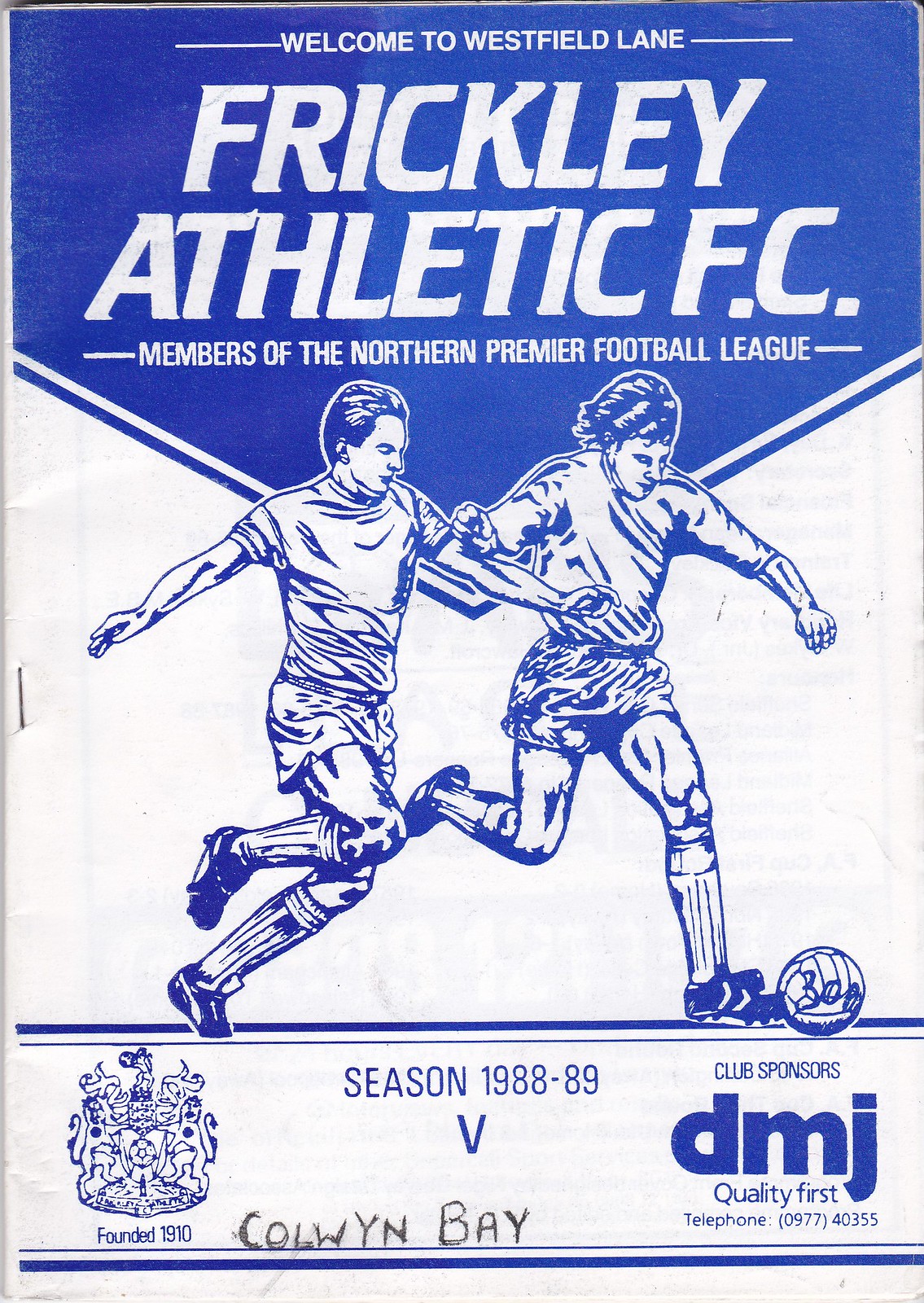The image is the front cover of a program for a soccer game, predominantly featuring blue and white colors. At the top, a blue banner with white text welcomes readers with "Welcome to Westfield Lane, Frickley Athletic FC," identifying them as members of the Northern Premier Football League. Below this, on a white background, are detailed blue outlines of two soccer players in action, each in uniform. Beneath the illustration, on the bottom left, is the club's crest with "Founded 1910." In the middle, it reads "Season 1988-89V." On the bottom right, it mentions the club's sponsors with "DMJ, Quality First," alongside a non-standard 10-digit phone number, indicating it might be international. Handwritten in black ink at the bottom center is "Colwyn Bay."